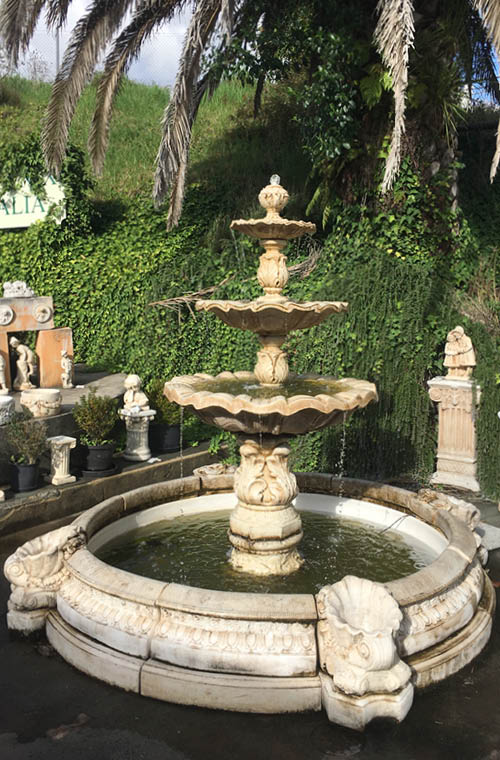The image captures a picturesque scene at a daytime tourist spot, possibly a park or garden, bathed in sunlight with a crisp blue sky in the background. Central to the photograph is a striking fountain constructed from pale stone, likely marble, featuring a main circular base adorned with intricate relief sculptures. Four levels make up the fountain: a wide circular basin at the bottom and three fluted, saucer-like tiers above, from which dark olive green water cascades downward.

Surrounding the fountain, a boundary wall and various white statuary, columns, and potted plants add to the old European aesthetic of the scene. To the left, a set of steps can be observed, leading to additional stone structures and smaller sculptures nestled among the foliage. In the backdrop, a small hilly area supports an incline densely covered with vines, and further back, palm trees with leaves and trunks entwined in vines frame the view. A signboard partially visible behind the fountain reads "ALIA". The dark gray stone ground contrasts with the abundance of greenery, creating a harmonious blend of natural and man-made beauty.